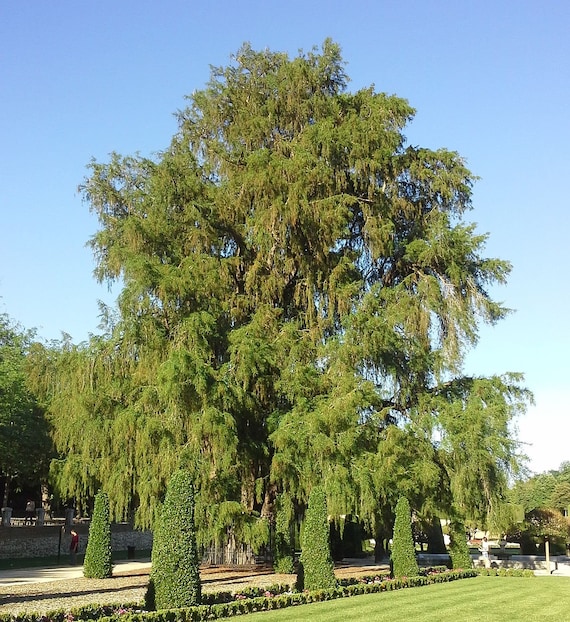This vibrant outdoor color photograph captures a stunning, well-manicured park on a beautiful, sunny day under a clear, blue sky. Dominating the background is a tall, majestic tree with lush green leaves, stretching up to the top of the image. In front of this grand tree, five meticulously trimmed, cone-shaped topiaries stand in a line, creating a formal and ornate foreground. The neatly maintained lawn is edged with smaller flowered plants and framed by a stone wall on the left. A few bystanders can be seen strolling along the gravel walkway, adding a touch of liveliness to this serene and picturesque park setting.